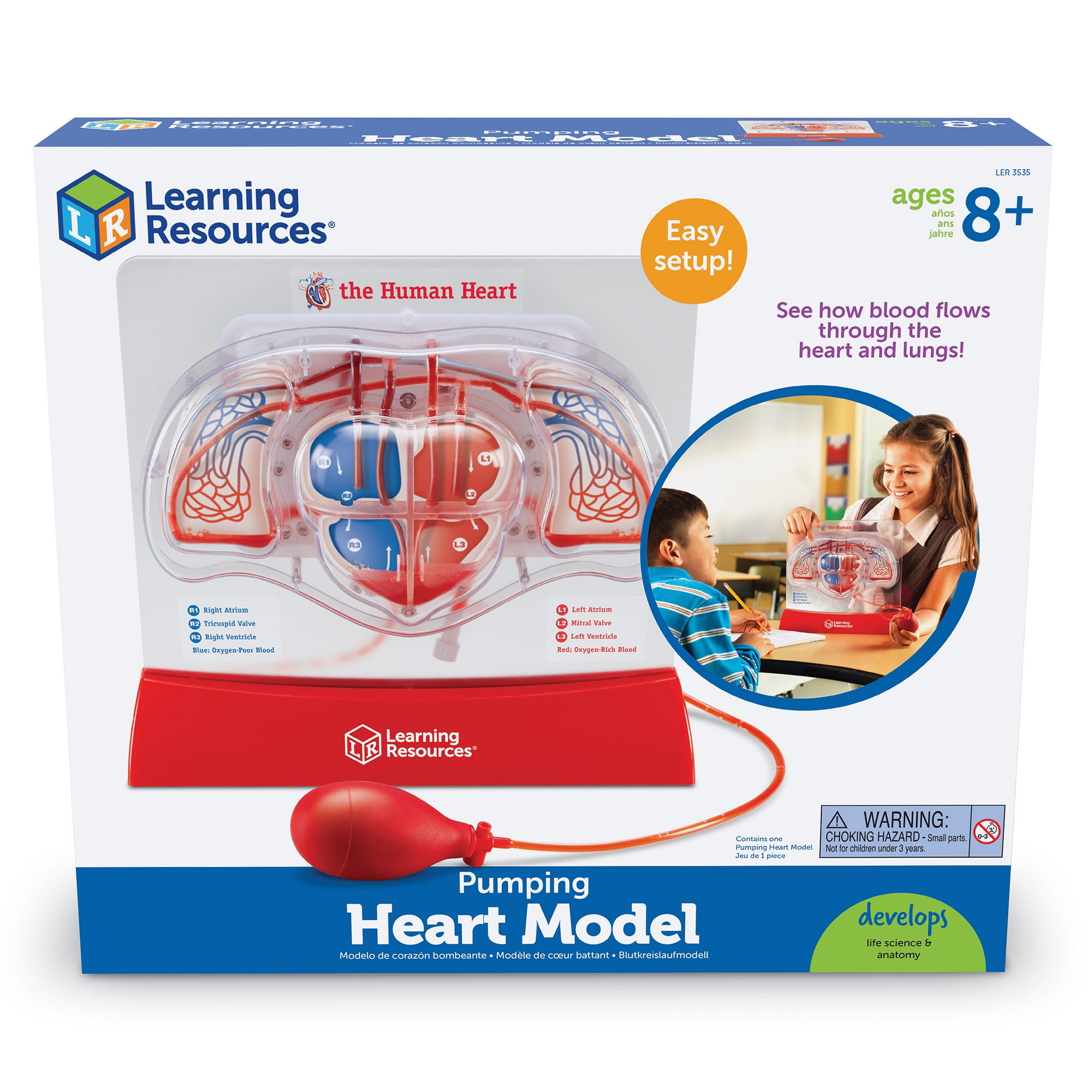The image depicts a box from Learning Resources, predominantly white at the top and blue on the left-hand side. The top left corner features a block with a green top and sides that are blue with a white "L" on the left and orange with a white "R" on the right. A blue banner at the bottom of the box reads "Pumping Heart Model" in white text. The box illustrates a toy human heart model, with the pump being red and the heart itself split into blue and red halves to distinguish the blood flow pathways. 

Upon zooming in, the left side of the heart is labeled as follows:
- L1: Left Arteries
- L2: Partially readable, ending in "Ralph"
- L3: Another term starting with "left"

The labels indicate that the red areas represent oxygen-rich blood. 

On the right side, the heart is labeled:
- R1: Right Atrium
- R2: Another partially readable word, potentially ending in "Ralph"
- R3: Begins with "Right"

The blue areas presumably represent deoxygenated blood. The text becomes blurry towards the bottom but likely includes the word "oxygen" and a further explanation about the blood's oxygenation status.